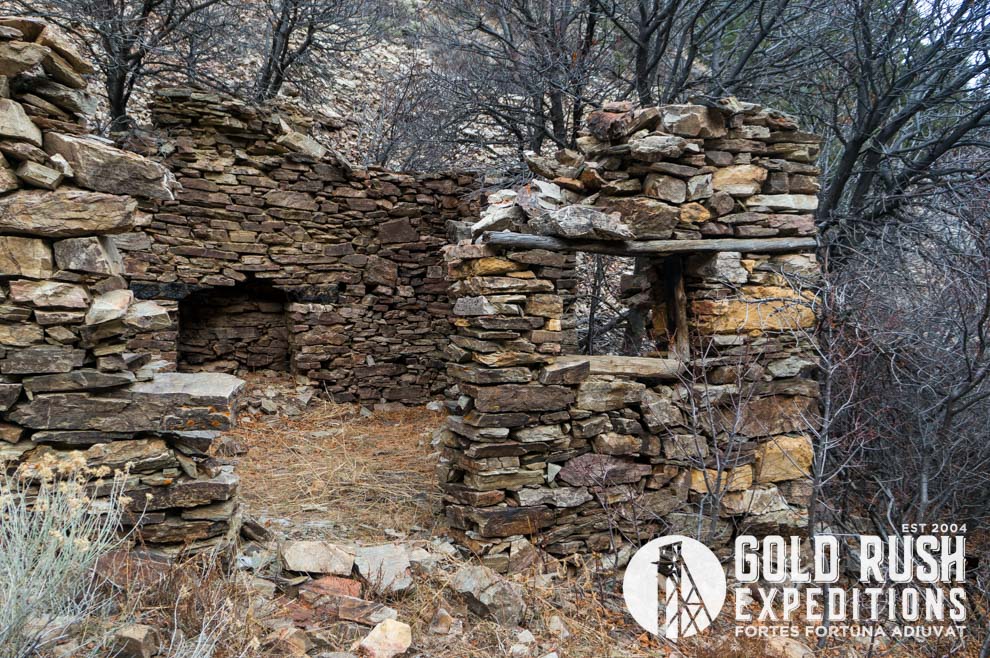This image, featured on a promotional brochure for Gold Rush Expeditions established in 2004, portrays a dilapidated ancient fort constructed from large, flat, rectangular rocks. The fort, now in severe disrepair, features four walls of varying integrity, lacking both a roof and door, which were likely once made of wood. To the right, a window cut-out reinforced by wood prevents the structure from collapsing entirely. In the far back wall, an indentation suggests the presence of a former fireplace. Surrounding the fort, leafless, brown trees frame the structure, suggesting a seasonal setting of either early spring or late fall, enhancing the desolate, historical atmosphere of the scene.